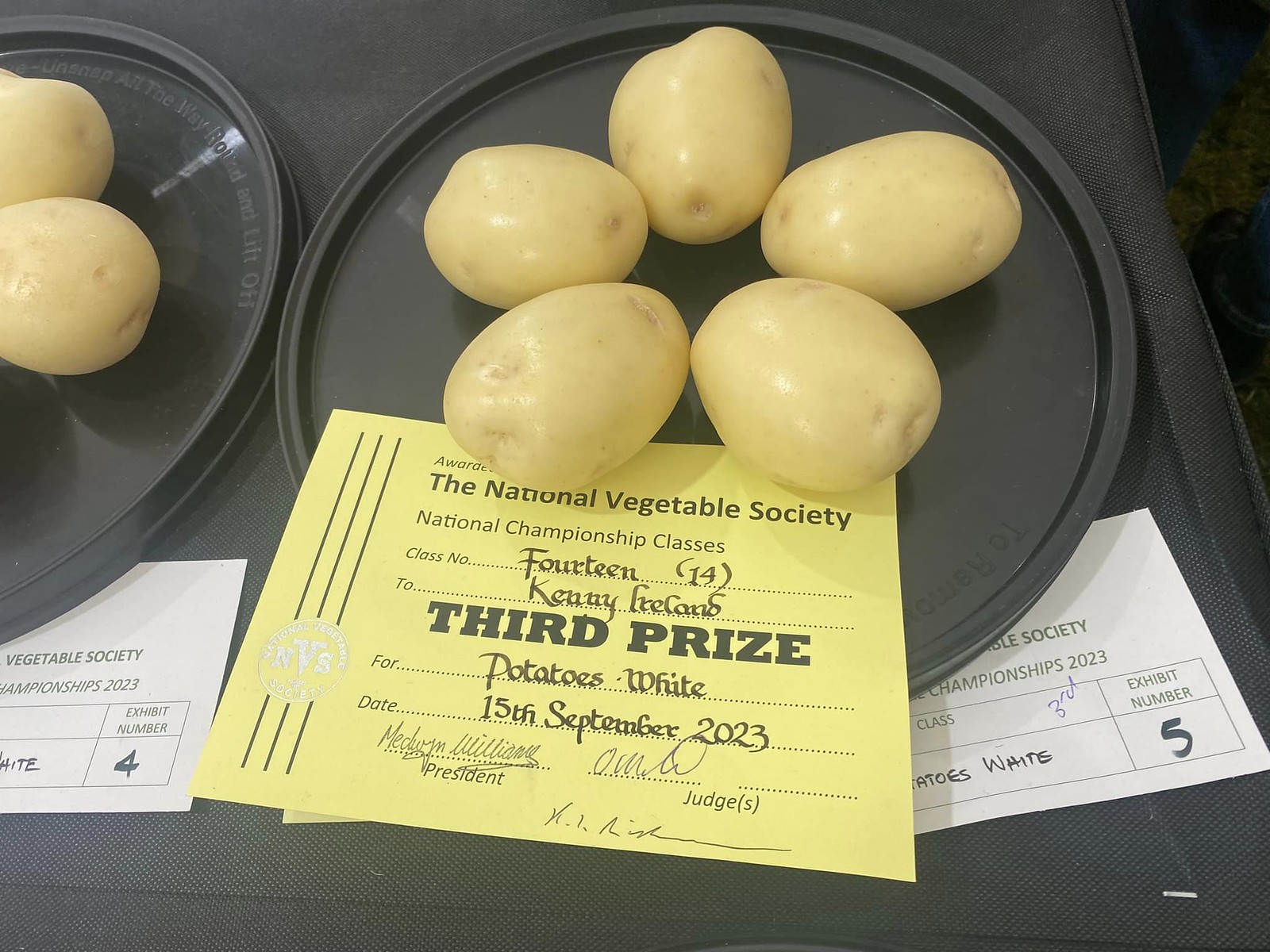The close-up image captures five neatly arranged potatoes on a black plate, which resembles the lid of a five-gallon bucket, all set on a black tabletop. To the left, part of another identically black-lidded plate is visible, holding two more potatoes. Positioned beneath the plate with the five potatoes is a yellow award certificate labeled "National Vegetable Society National Championship Classes, Class Number 14," and details a third prize win for "Potatoes-White," awarded to Kenny, Ireland, on the 15th of September, 2023. The certificate, adorned with signatures from both the president and judges, lends an air of formality to the scene. The entire setting is brightly lit, highlighting the contrasting colors and creating a vivid visual of the proud display.